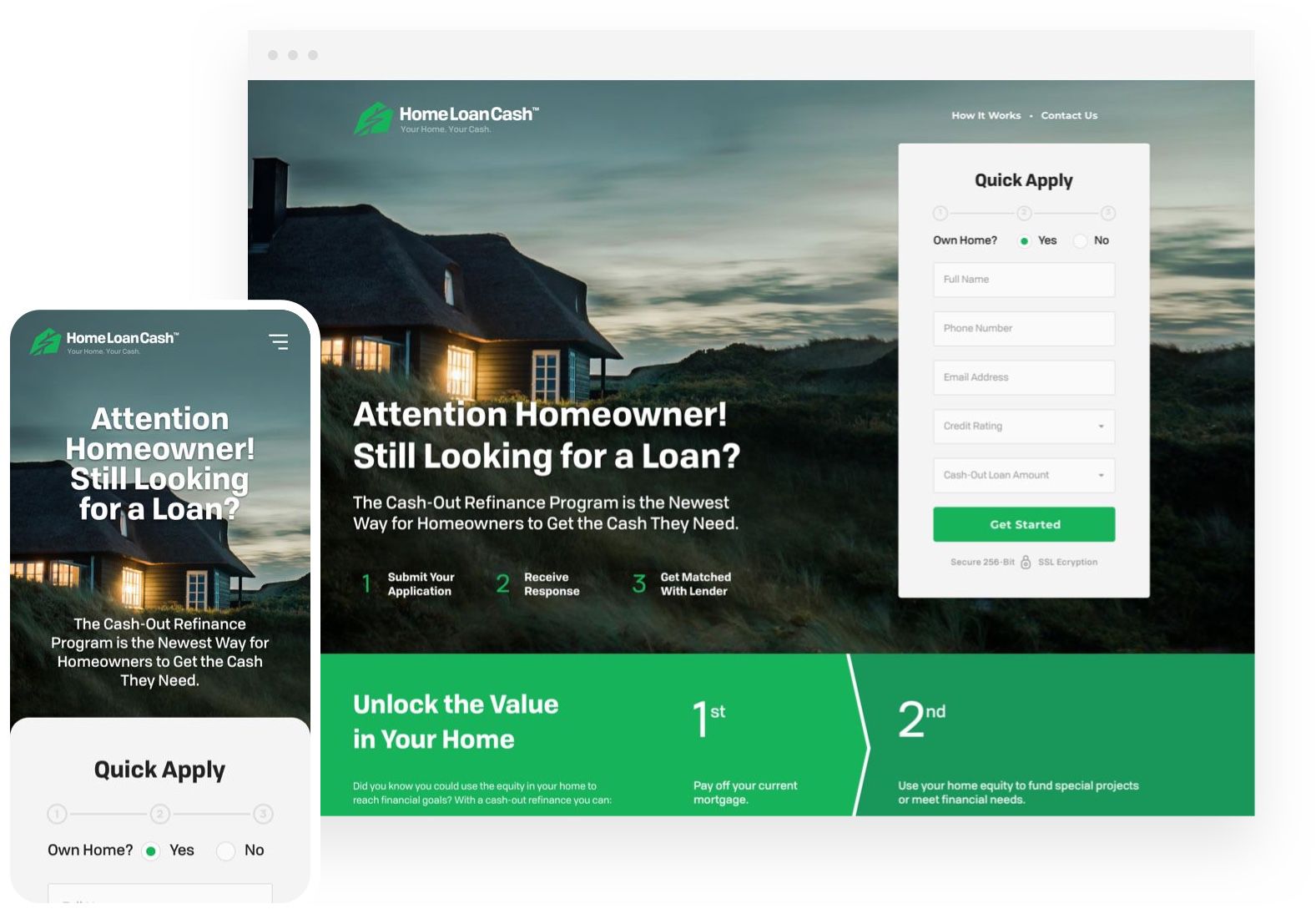This is a detailed screenshot of a web page and a phone interface for a website called "Home Loan Cash." The tagline under the website's name reads "Your Home, Your Cash," accompanied by a green business symbol to the left. Both the desktop and mobile versions display an image of a house with a distinctive curved dark roof and typical dark siding. White-framed windows brightly illuminate the home, which is set against the backdrop of a field with tall grass in the foreground and a slight hill to the right.

Text on both platforms reads: "Attention Homeowner: Still looking for a loan? The cash-out refinance program is the newest way for homeowners to get the cash they need." The mobile app features a "Quick Apply" section asking "Own Home?" with options for "Yes" or "No," and "Yes" highlighted.

The laptop website lists a streamlined three-step process: 
1. Submit your application.
2. Receive a response. 
3. Get matched with a lender.

Additional text explains: "Unlock the value of your home. First, pay off your current mortgage. Second, use your home equity to fund special projects or meet financial needs." An inset box on the web page contains the "Quick Apply" form, which asks for personal details such as phone number, name, and credit rating.